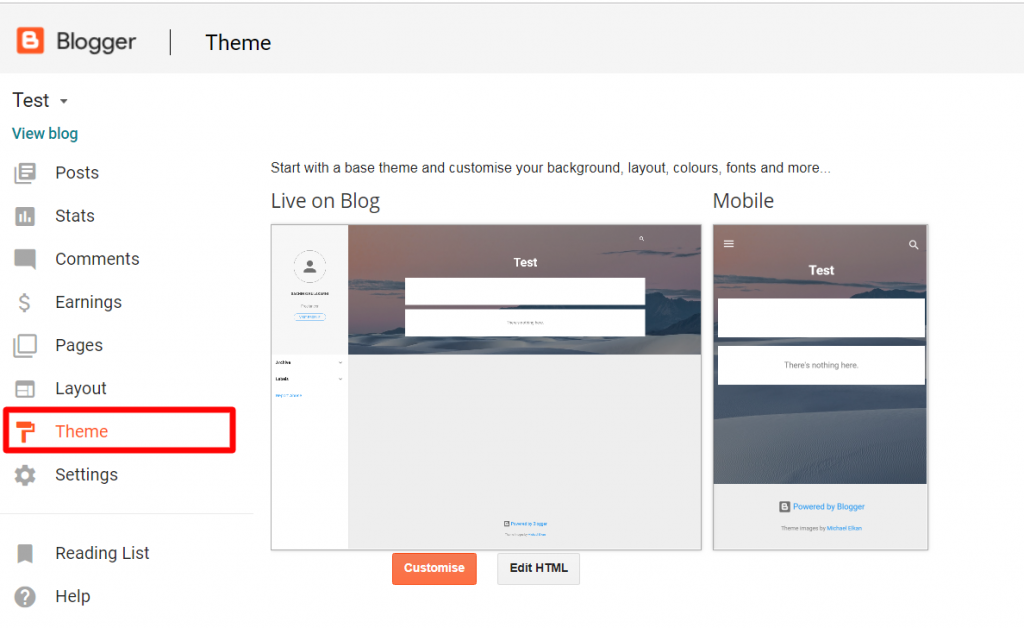In this detailed image of a Blogger website interface, we start with the top left corner where the word "Blogger" is displayed prominently. To the right, under a light gray background that stretches across the screen, are the words "Theme," "Test," and "View Blog." 

On the left sidebar, various categories are listed vertically: 
- Posts
- Stats
- Comments
- Earnings
- Pages
- Layout
- Theme (highlighted with a bright red rectangle and displayed in orange text)
- Settings
- Reading List
- Help at the bottom 

On the right side of the image, a screen displays a sentence at the top that reads: "Start with a base theme and customize your background, layout, colors, fonts, and more." 

The left-hand side of this section labeled "Live on blog" features a preview design of the blog, labeled "Test," with two white rectangles set against a light gray background. The header region above the background blends shades of purple, black, and gray. On the right side is a mobile version preview, also labeled "Test," showing a similar, smaller screen design.

At the very bottom of this section, there is an orange rectangle labeled "Customize" next to a light gray rectangle that reads "Edit HTML." The entire interface is surrounded by a light gray or white background, providing a clean and structured look.